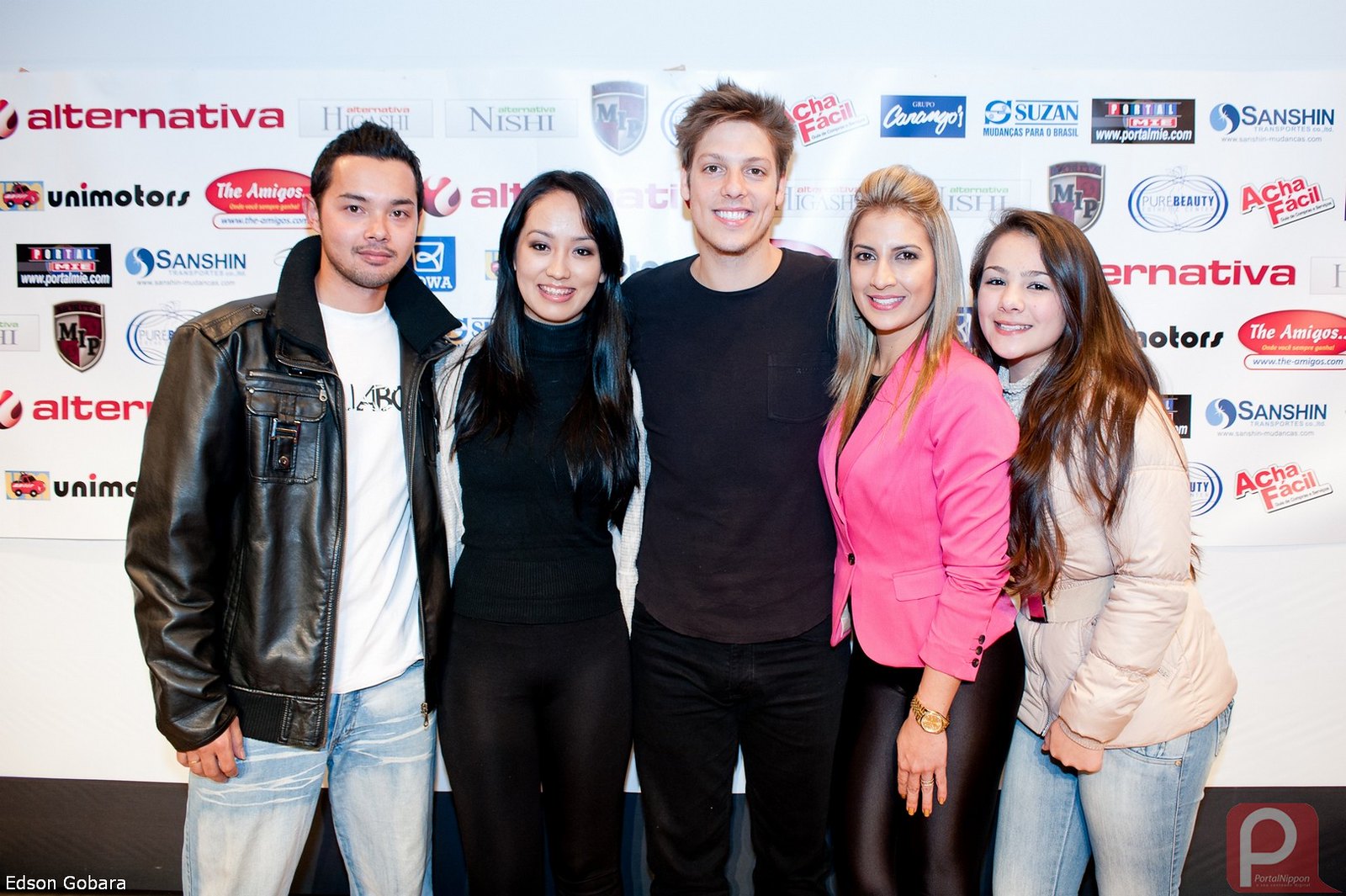In the image, five young individuals are posing in front of a backdrop adorned with various sponsor logos such as Alternativa, Susan, Sanxing, and Achi Fasi, repeated frequently. From left to right, the group consists of:

- A young Asian man with a clean short haircut, wearing a black leather jacket over a white t-shirt and blue jeans.
- An Asian woman with long, shiny black hair, dressed in a tight-fitting black turtleneck and tight black leggings, paired with a white jacket.
- A taller white man with brown hair, styled full on top, donning a purple t-shirt with a pocket and black jeans.
- A blonde woman with light skin, wearing a short pink jacket and very tight black leggings that appear leathery.
- A younger woman with long reddish-brown hair, in a cream-colored sweatshirt and blue jeans.

They are aligned in front of the backdrop in a style reminiscent of a photo shoot.